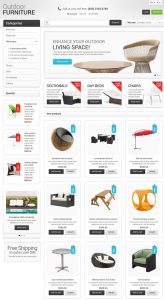This image depicts a website dedicated to selling outdoor furniture, although the quality of the image makes much of the text difficult to read. In the upper left-hand corner, the text “Outdoor Furniture” is visible, followed by a series of illegible words. The center of the page features the text “Your Outdoor Living Space” and showcases images of various outdoor products available for purchase. 

Notable items include a bird bath in a natural color, along with what seems to be a chaise lounge, and a white table, although these pictures are also quite blurry. Additional images display what appears to be different kinds of seating options and a table surrounded by chairs. There is also an image of an umbrella and several more pictures of chairs, including a black outdoor loveseat, and a picnic table. Another image showcases a yellowish-orange outdoor item. Near the bottom, there is a whitish-gray table and another type of seating. The final image features a black chair with a cushion. Despite the blurriness, the assortment indicates a wide range of outdoor furniture options available on the website.